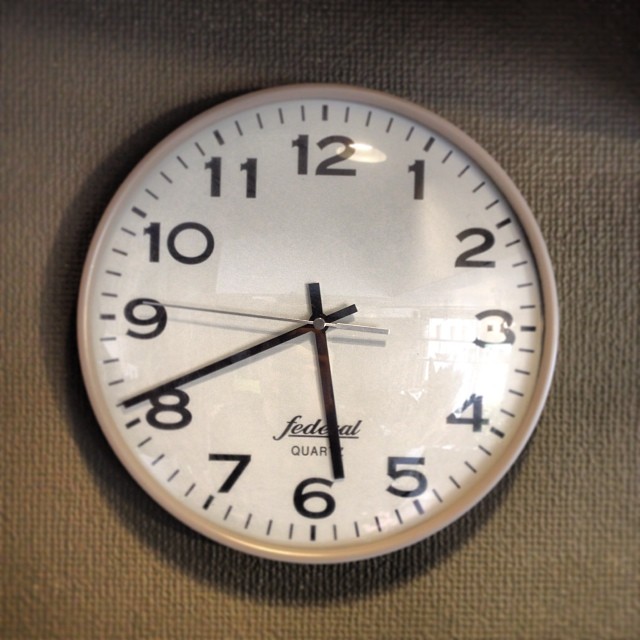The image features a wall clock set against a textured brownish-gray background with a fabric-like or wallpaper appearance, accentuated by shadows. The clock itself has a sleek silverish-white outline, with standard Arabic numerals from 1 to 12 around its face, marked in black, with the number 12 at the top and 6 at the bottom. Below the number 6, the text "federal quarry" is prominently displayed, with "Federal" underlined. The clock's short hand is positioned between the numbers 5 and 6, while the long hand is pointing just past the 8.